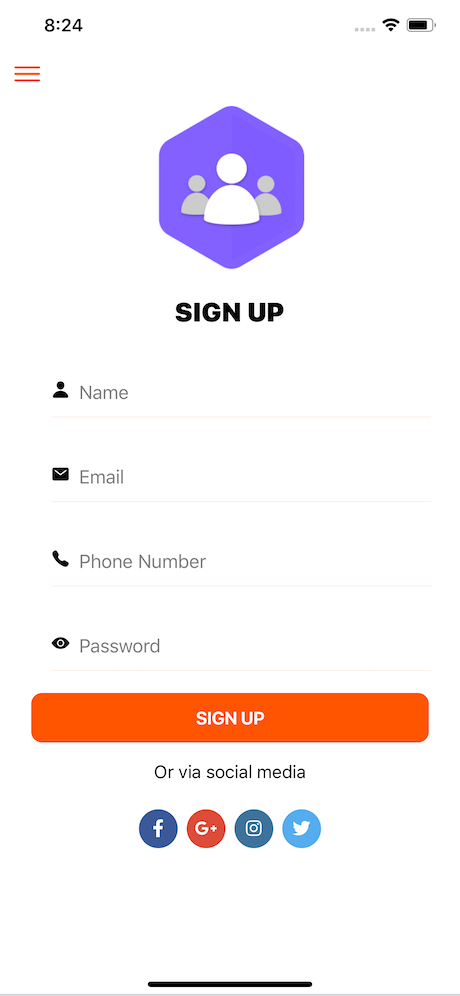This image captures a screenshot of a sign-in page for an app or website on a mobile device, displayed in a vertical orientation. The device indicates the time as 8:24 AM in the top left corner. In the top right corner, the battery icon shows approximately 80% charge. The Wi-Fi icon is solid black, accompanied by four gray dots arranged horizontally.

Beneath the time, three horizontal red lines, parallel to each other, are visible. Dominating the center of the screen is a purple hexagon logo, below which are three icons depicting stylized human figures. The first icon is a white circle for the head atop a white half-circle for the body, with two similar icons in gray positioned behind it to the left and right.

Prominently displayed below the icons is a black bold and capitalized text reading "SIGN UP." Below this header, a series of input fields are arranged vertically. These fields are labeled as "Name," "Email," "Phone Number," and "Password." Underneath the input fields lies a large orange rectangular button with the text "SIGN UP" in white, uppercase letters.

At the bottom of the screen, the text "or via social media" precedes four circular icons that represent Facebook, Google Plus, Instagram, and Twitter.